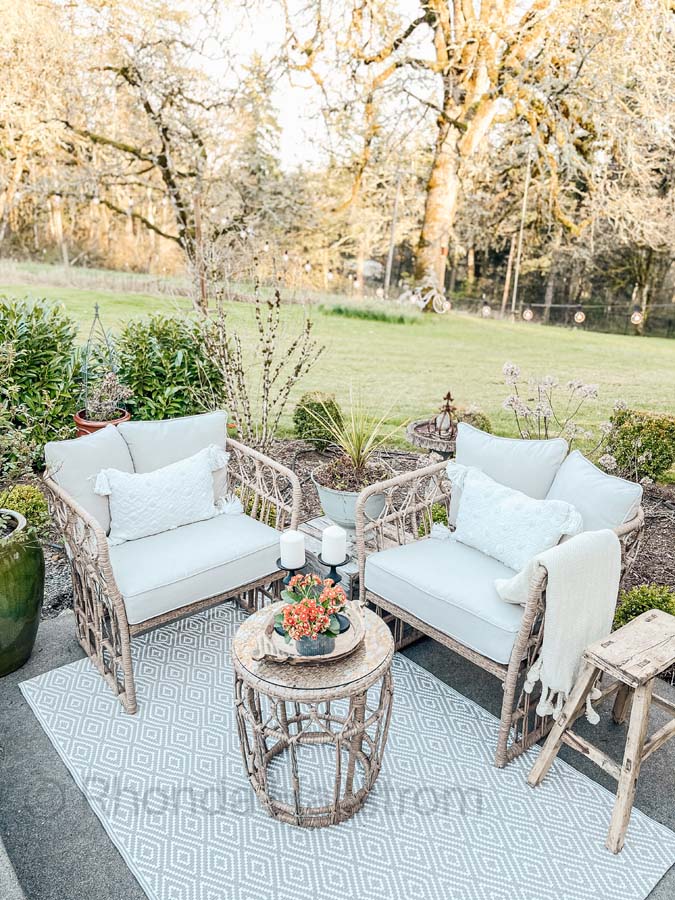This detailed vertical color photograph captures a beautifully designed patio set in a serene outdoor setting. The patio features stylish wicker furniture adorned with white and mint-green cushions, creating a cozy and inviting atmosphere. The seating area includes two cushioned chairs and a small round wicker coffee table topped with orange plants arranged on a tray. 

Complementing the chairs is an additional side table, creatively repurposed from a bench, positioned between them. The patio is adorned with a green patterned rug, adding a vibrant touch underfoot. Surrounding the seating area, black candle holders with candles add a touch of elegance.

In the background, mature trees and a well-manicured lawn, reminiscent of a golf course, enhance the tranquil ambiance. Twinkle lights are strung above, poised to cast a charming glow when night falls. Nearby, a motorcycle is subtly parked beside a tree which also bears a red sign, adding a hint of curiosity to the scene.

Ensuring the vibrant setting, various flowers, including Queen Anne's lace and spider plants, are meticulously planted around the patio area, creating a lush, well-tended garden that completes this picturesque outdoor retreat.